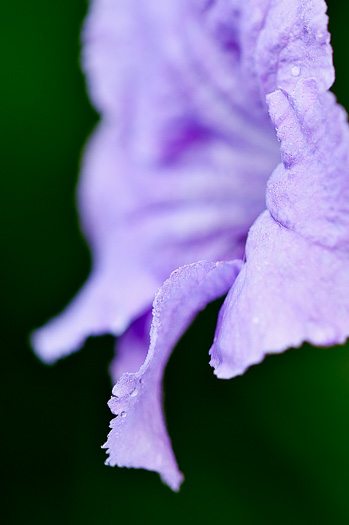In a dimly lit setting, a meticulously captured photograph draws attention to the intricate details of a purple flower. The professional lighting casts a gentle glow that highlights the edge of a dew-kissed petal. The focus is razor-sharp on the serrated edges of the petal, revealing tiny droplets of moisture clinging to its surface. In the blurred background, a bell-shaped flower with pronounced striations emerges, providing a textured contrast against the dark backdrop. The composition leads us to imagine accompanying leaves and a stem, all softly out of focus. Fine veins weave across the petals within the scene, giving depth to the floral subject facing towards the left. The artistry in the lighting, angle, and focus invites us to appreciate the delicate beauty and complexity of this botanical marvel.